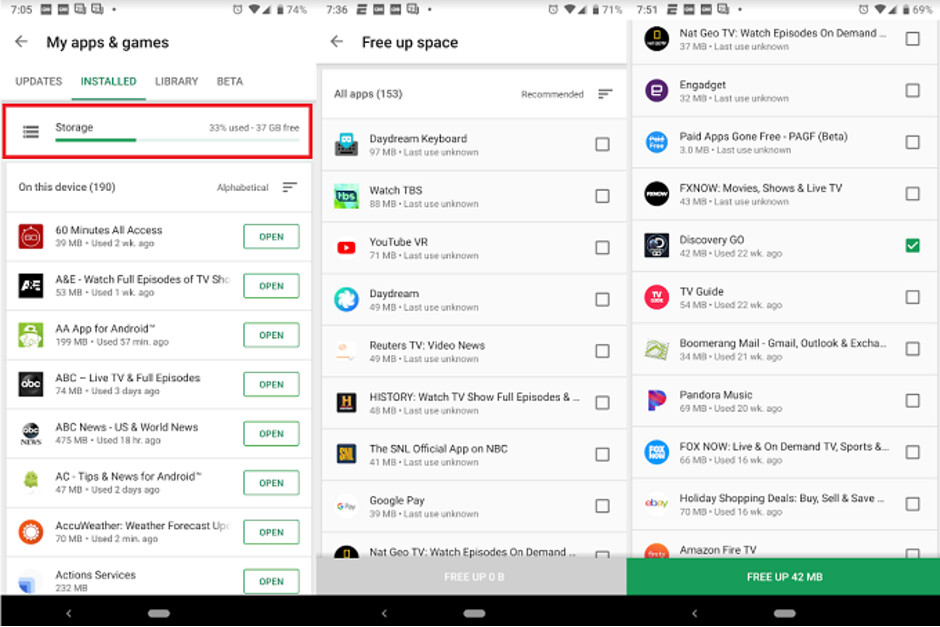The image is a compilation of smartphone interface screenshots, arranged in a row. Each screenshot features a black navigation bar at the bottom, containing a small oval "Back" button on the left and a "Home" button. At the top, there is a status bar displaying the time, various phone icons, and battery life indicators.

The far-left screenshot is titled "My Apps & Games" and displays the "Installed" tab highlighted. Various installed apps are listed under this tab.

The center screenshot focuses on the "Free up space" option, positioned below the top status bar. It lists several apps with checkboxes next to each, indicating they can be selected for removal to free up space.

The far-right screenshot, still within the "Free up space" interface, shows a scrolled-down view where one of the apps has been selected and highlighted. The "Free up" button at the bottom is now active and ready to be tapped.